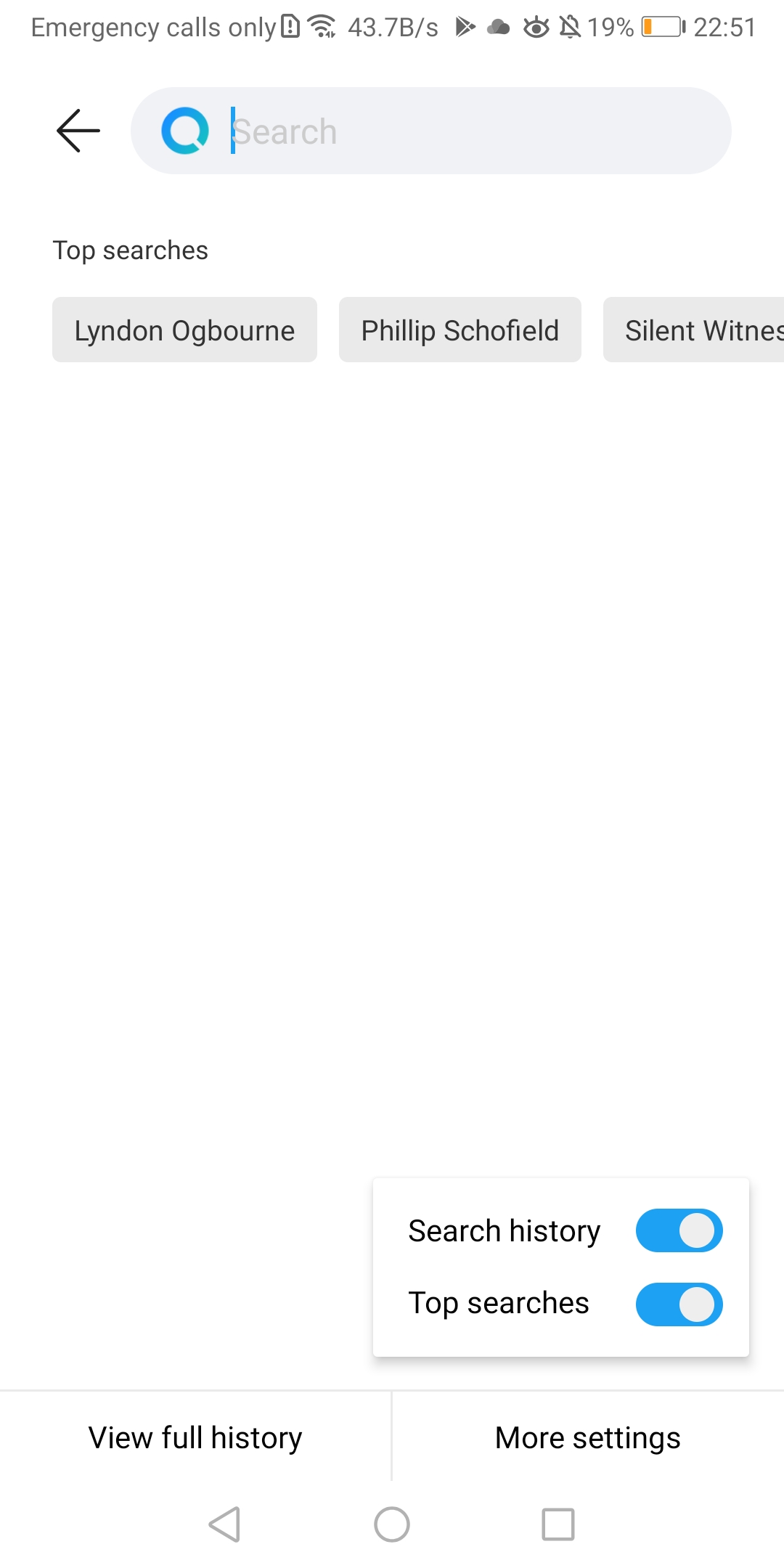**Caption:**

A mobile device screenshot displaying the search interface. At the top, a search bar is prominently featured. Below the search bar is a label titled "Top Searches," listing three popular queries: Lyndon Ogburn, Philip Schofield, and Silent Witness. The majority of the screen is occupied by a large white space. Near the bottom, there are two toggles labeled "Search History" and "Top Searches," both in the "on" position. At the very bottom of the screen, options for "View Full History" and "More Settings" are available for further user interaction.